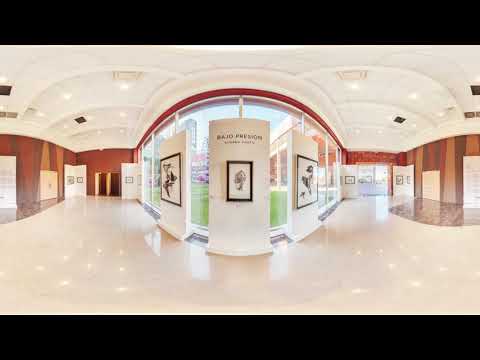The photograph, likely taken with a fisheye or 360-degree lens, captures an indoor setting that could be an art gallery or modern lobby. The image is bordered by black horizontal bars at the top and bottom, reinforcing its panoramic nature. The bright, reflective white floor contrasts with the white ceiling, which features darker squares, possibly vents. The room's walls are a rich mosaic of brown wood panels, adding warmth to the space. A series of tall, white rectangular pillars stand in front of large, curved windows, distorted by the unique lens. These pillars display framed photographs or artwork, each set in black frames with white mats, potentially showcasing floral designs. The scene is brightly lit, suggesting daylight streaming through the expansive windows, which also offer views of doorways leading outside. The overall image exudes a modern, airy feel, with abundant natural light enhancing the gallery-like ambiance.